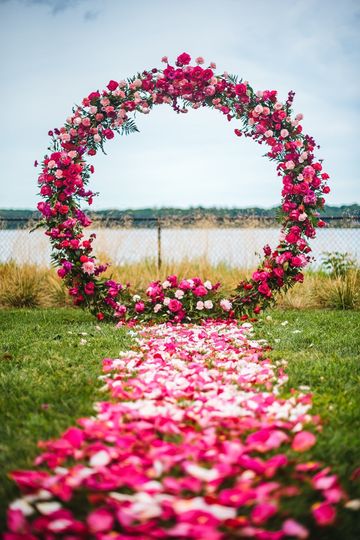The photograph captures an outdoor scene set up for a wedding, featuring a lush, green field with a striking circular, floral wreath that acts as an altar. The wreath, approximately six to eight feet in diameter, is adorned with an array of vivid pink, red, and white roses, with some flowers in light pink and the majority in a deep, dark pink. These blooms are complemented by a backdrop of green foliage, contributing to the wreath's opulent appearance. 

Leading up to this ornate structure is a rectangular path made of scattered pink flower petals, forming a vivid and romantic trail that stretches 10 to 15 feet across the grassy field. The setting includes marsh grass interspersed within the main grassy area, adding to the natural, earthy feel of the scene. 

Behind the wreath, beyond a chain link fence with metal posts, lies a large, serene body of water, possibly a lake, with its calm, gray surface reflecting the overcast sky above. The horizon features a mix of low-lying vegetation and dark green hills, set against a predominantly cloudy, moody gray sky that suggests a humid atmosphere. This picturesque scene, rich with detail and natural beauty, seems perfectly orchestrated for a wedding ceremony.